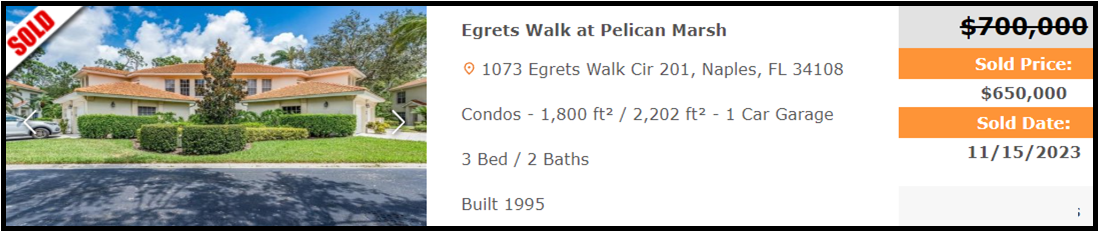This screenshot showcases a real estate listing for a recently sold property in Naples, Florida, situated at 1073 Egeritz Walk Circle, Unit 201, in the 34108 ZIP code. This property comprises attached condos or townhouses located in a cul-de-sac within Pelican March. Featured in the image is a well-maintained residence constructed in 1995, painted green, and boasting a neatly manicured front yard. The living space ranges between 1,800 to 2,200 square feet and includes three bedrooms, two bathrooms, and a one-car garage. The property sold for $650,000 on November 15, 2023, down from its original list price of $700,000. The photograph captured on a day with a partly cloudy, blue sky also includes a white car parked in the driveway with a prominent "SOLD" sign superimposed over the image.